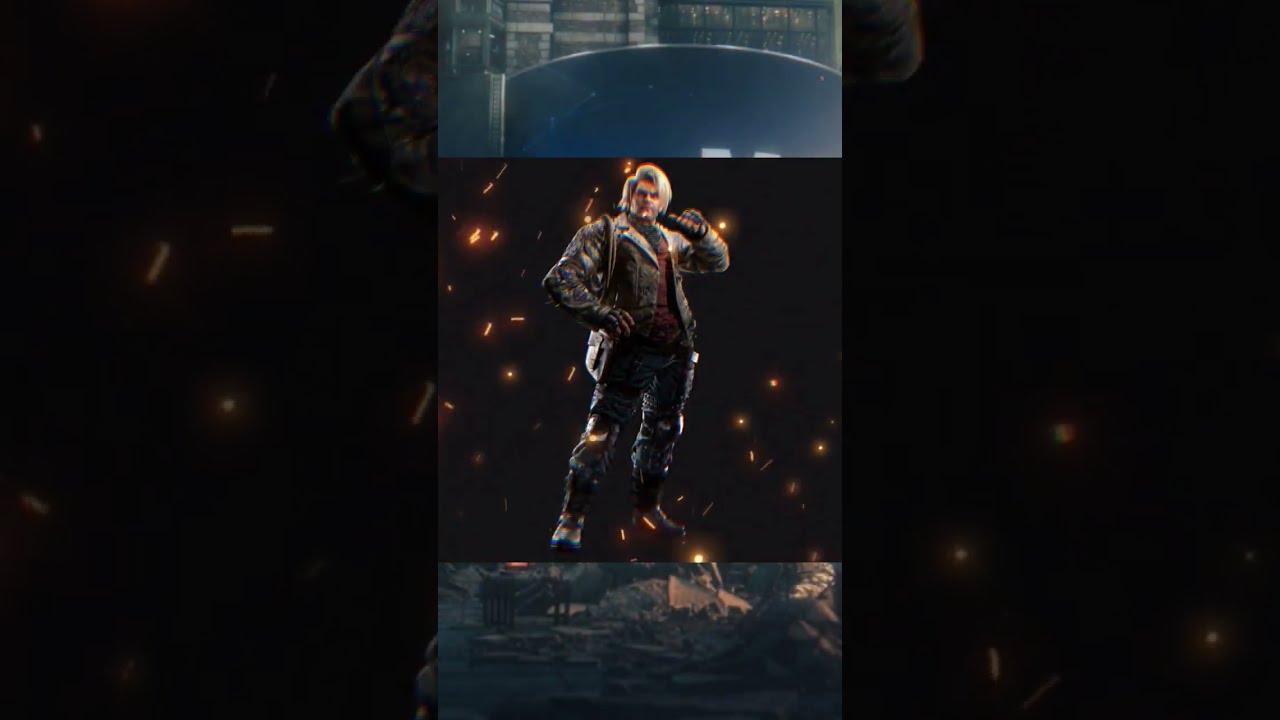The image is an illustration resembling a video game screenshot of a male character positioned centrally. He is shown facing the viewer, holding a microphone—or possibly a weapon—in his left hand. Dressed in a combat uniform comprising a black army coat, dark black pants, black gloves, and boots, he also has a red shirt underneath and a bag slung over his right shoulder. The character has medium-length blonde hair. The background spans three vertical rectangles filled with a dark, black color adorned with orange and whitish sparks or dots, giving a starry night effect. The top portion of the image includes indistinct, bluish elements, adding to the atmospheric tension. Below the character, the ground appears to be rubble, hinting at a war-torn or distressed setting.